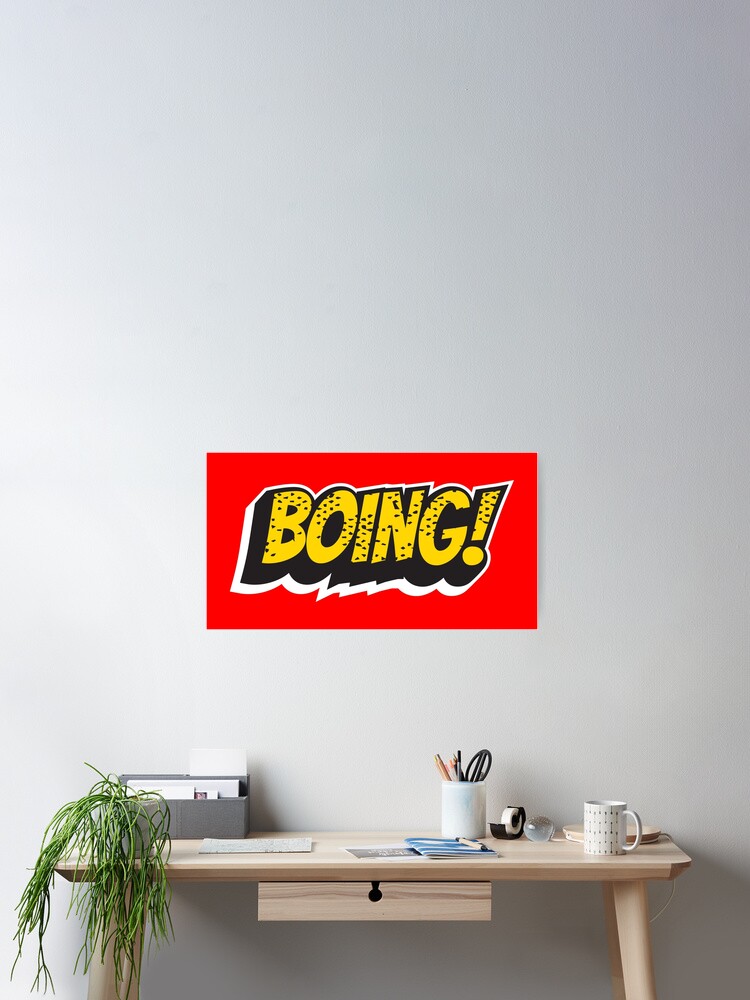This image showcases a section of a room, focusing on a small, light-colored wooden desk positioned against a plain white wall. Dominating the wall above the desk is a simple, eye-catching poster with a red background and large yellow cartoon text, outlined in black shadow and white highlights, that reads "Boing." 

The compact desk features a small drawer attached to its underside, adding a touch of functionality. To the left side of the desk, there is a green house plant with drooping leaves that extend below the desk surface slightly. Behind the plant sits a small organizing container and a piece of paper. On the right side, the desk hosts a collection of common office supplies, which include a lamp, a mug, another cup holding pens and scissors, and a roll of tape. Additionally, there is a protractor and a book, further emphasizing the workspace's practical use. This detailed arrangement creates a tidy and organized yet functional atmosphere ideal for work or study.